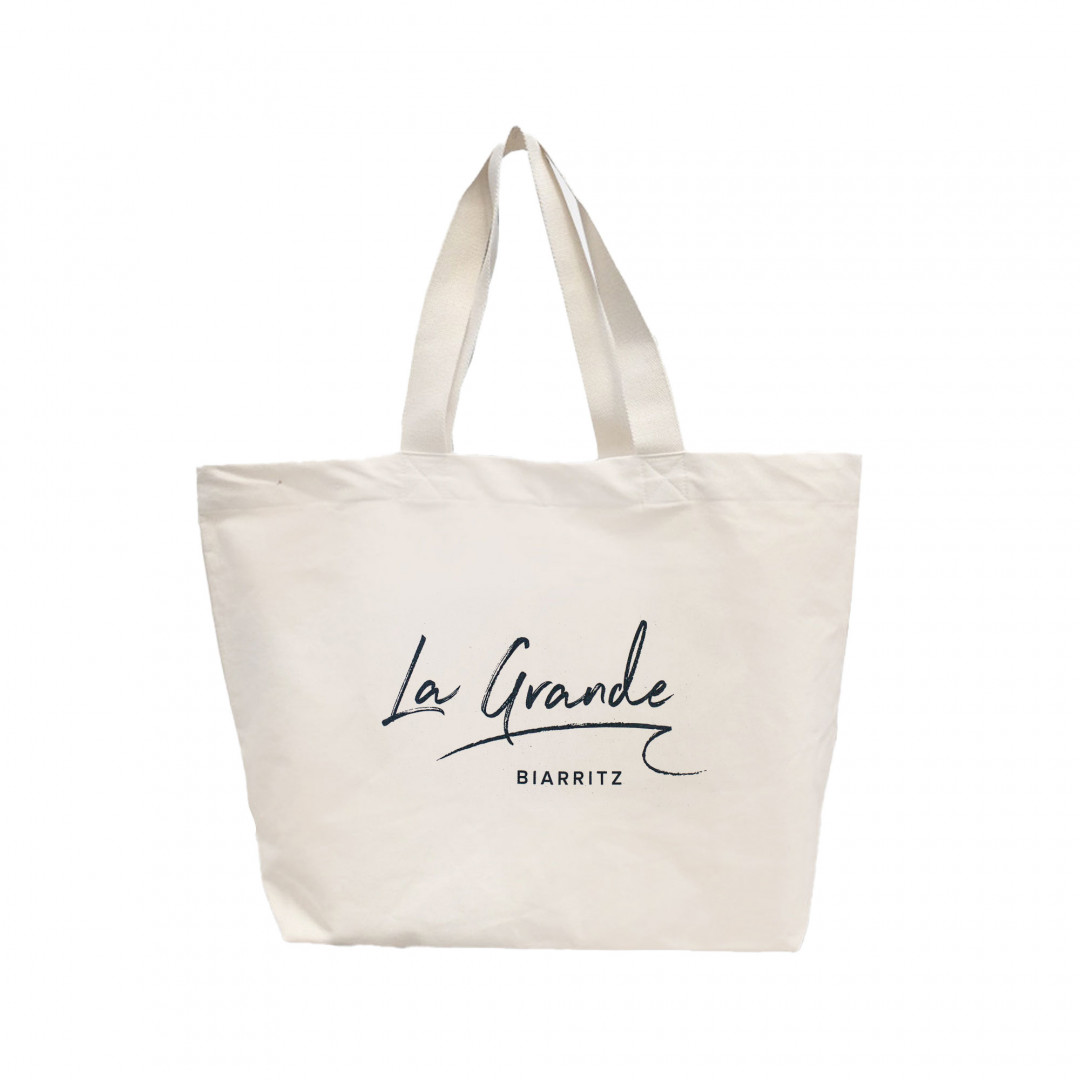The image features a reusable tote bag crafted from white canvas material, standing upright against a pure white background. The bag showcases a simple yet elegant design with two handles seamlessly attached at the top, highlighted by X-marked white stitching. The bag's off-white, beige hue adds to its minimalist charm. Prominently displayed in the center, the text "La Grande" is written in black cursive font with an accentuated underline extending beneath it, followed by the word "Biarritz" in a plain, blocky typeface. The tote bag, medium-sized with a trapezoidal shape, embodies practicality and style, making it a versatile accessory likely to hold numerous items.